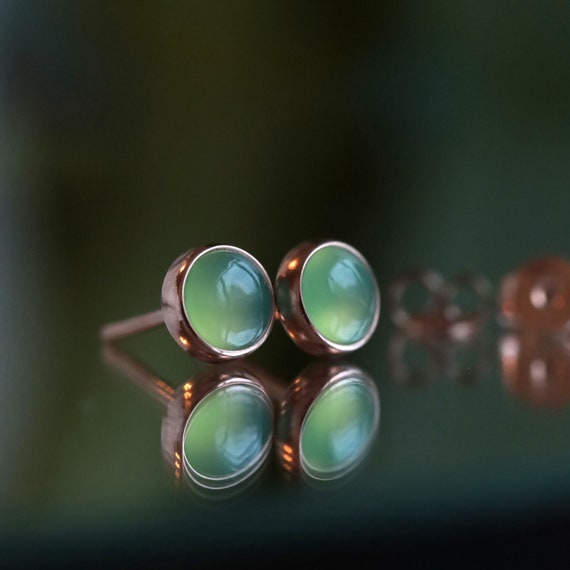A square photograph features a stunning display of jewelry against a dark green backdrop adorned with subtle, lighter green lines, likely reflections from the jewelry itself. The focus is on a pair of elegant emerald earrings, encased in gold bands. These earrings are positioned horizontally, side by side, in the center of the image, their reflections clearly visible at the bottom. To the right, another set of green-hued earrings is partially visible, positioned towards the middle of the frame. Surrounding these primary pieces, the out-of-focus image reveals additional gold and coppery metallic jewelry, adding a rich, luxurious depth to the scene.